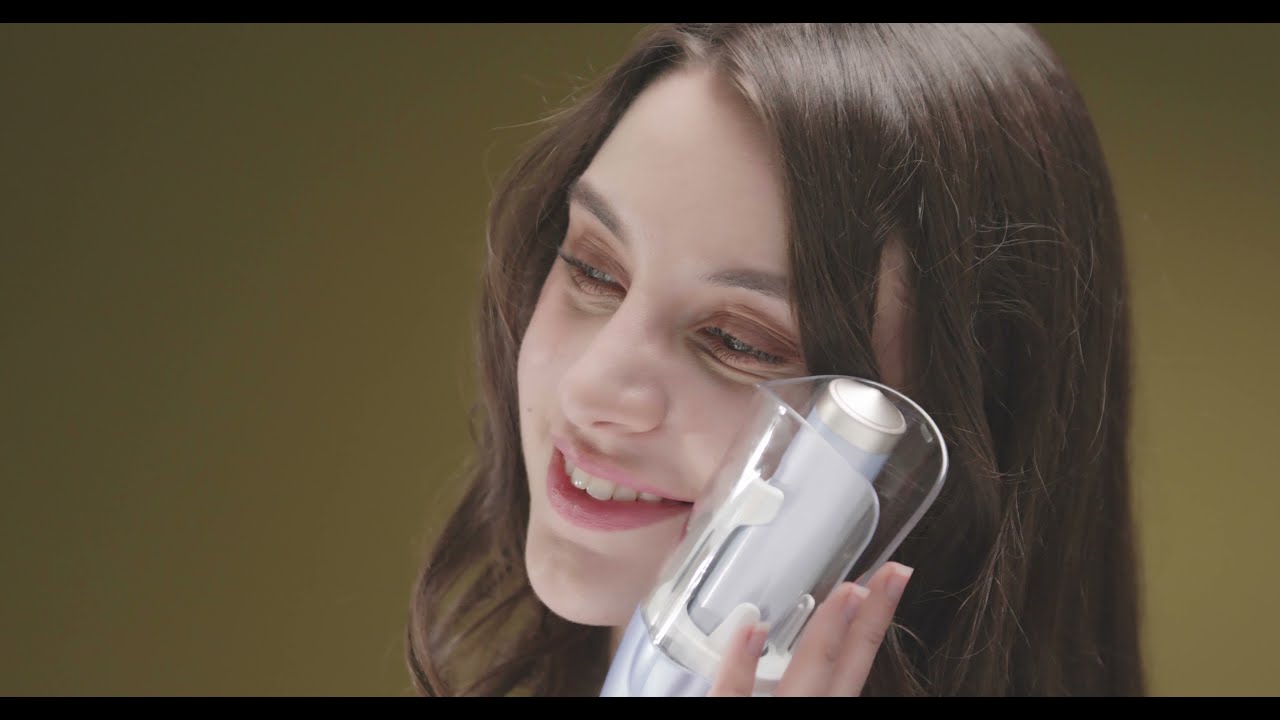This is a well-lit, studio-photographed image of a smiling Caucasian woman with smooth skin and long, flowing brown hair. She has greenish eyes and pink lips, with her partially closed eyes showing bags underneath, possibly enhanced by light brown eyeshadow. Her eyebrows appear neat and trimmed. The woman is leaning towards a cylindrical, light purple, silver, and clear plastic device, which she is holding up to her cheek, suggesting it might be a beauty product. Her head is slightly tilted, and she seems to be looking downwards to the left side of the frame. She is wearing natural makeup and has long nails. The background showcases a gradient of brown shades, shifting from darker to lighter areas, with black borders at the top and bottom of the image.